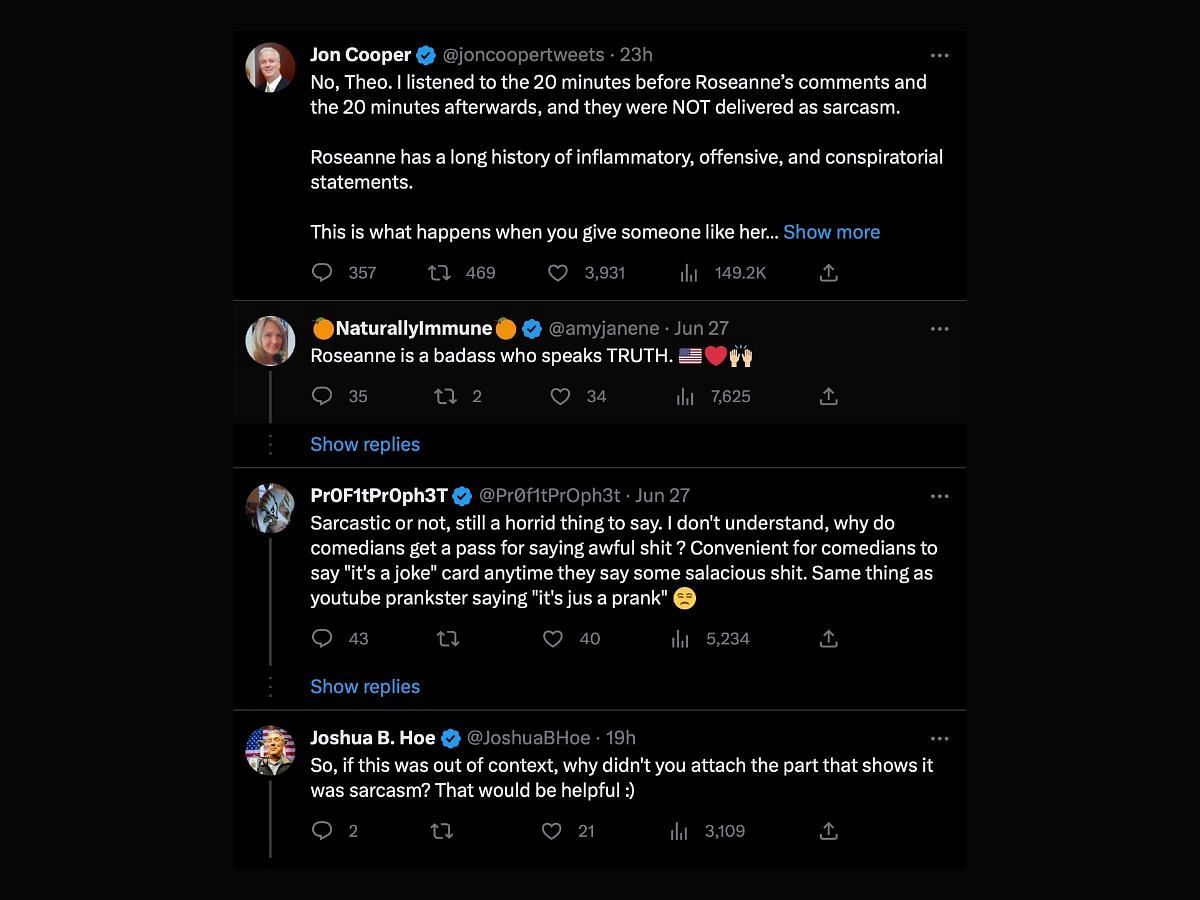The image is a screenshot of a Twitter conversation set against a jet-black background, displaying four posts from users John Cooper, Naturally Immune, P-R-O-F-1-T P-R-O-P-H-3-T, and Joshua B. Ho. 

John Cooper initiates the conversation, stating: "No, Theo, I listened to the 20 minutes before Roseanne's comments and the 20 minutes afterwards and they were not delivered as sarcasm." This post includes icons at the bottom indicating the number of likes, reshares, comments, views, and an up arrow for additional interactions.

Naturally Immune replies with: "Roseanne is a badass who speaks truth," accompanied by three icons representing social media interactions.

A gray line separates this post from the next, where P-R-O-F-1-T P-R-O-P-H-3-T writes: "Sarcastic or not, still a horrid thing to say. I don't understand why comedians get a pass for saying awful shit." 

Underneath, Joshua B. Ho questions: "So if this was out of context, why didn’t you attach the part that shows it was sarcasm? That would be helpful.”